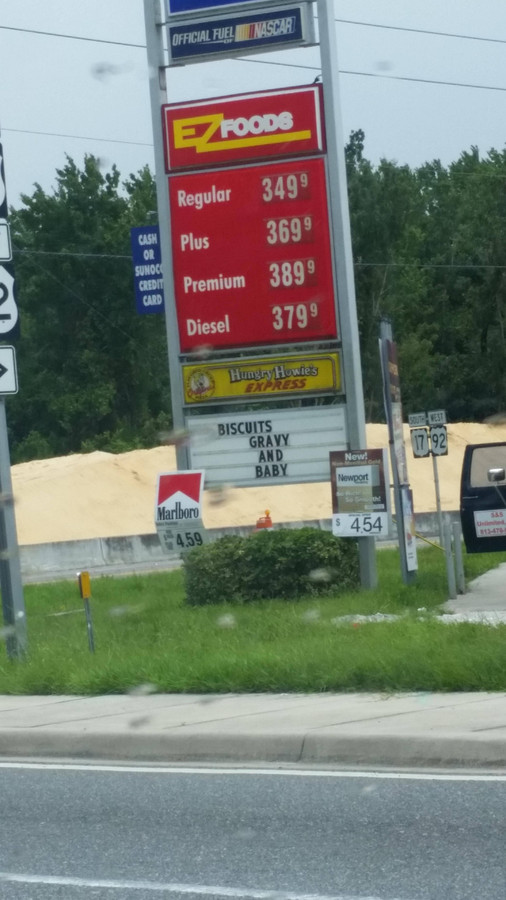In this outdoor daytime photo, we are standing on the road, gazing across to the other side of the street. Dominating the scene is a large, multi-tiered gas station sign situated in a grassy area. The sign is held up by two gray poles and features the text "Official Fuel of NASCAR" and "Easy Foods." Displayed prominently in red, the gas prices are as follows: regular $3.49.9, plus $3.69.9, premium $3.89.9, and diesel $3.79.9. Below the red sign, a yellow sign advertises Hungry Howie's Express. At the bottom of the sign, a white marquee with black letters promotes "Biscuits, Gravy, and Baby." The overall lighting is daytime but appears somewhat dim.